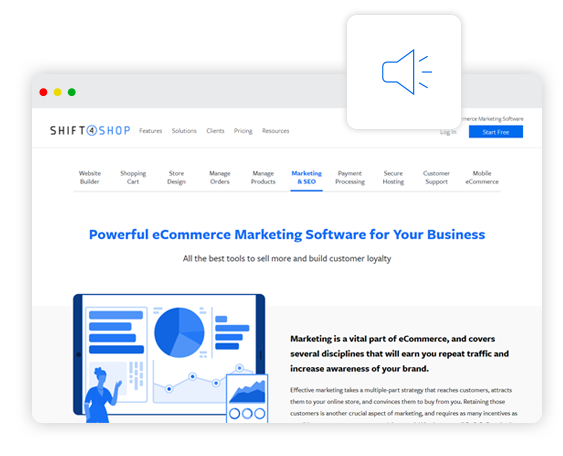Here's a cleaned-up and detailed caption for the image:

---

This is a screenshot from my website, Shift4Shop, showcasing our powerful e-commerce marketing software designed to elevate your business. The interface features a navigation menu in the upper left corner with three colored dots: red, yellow, and green, representing the window control buttons. Below, the menu options include "Features," "Solutions," "Clients," "Pricing," and "Resources" for easy access to various sections of the website.

Additionally, there are comprehensive links for essential tools and functionalities, including "Website Builder," "Shopping Cart," "Store Design," "Manage Orders," "Manage Products," "Marketing and SEO," "Payment Processing," "Secure Hosting," "Customer Support," and "Mobile E-commerce." A prominent "Start Free" button encourages new users to begin their journey, alongside a "Login" option for returning users.

Shift4Shop integrates all the best tools to help you sell more products and build lasting customer loyalty. Our platform highlights the critical role of marketing in e-commerce, encompassing multiple disciplines to drive repeat traffic and boost your brand's visibility.

---